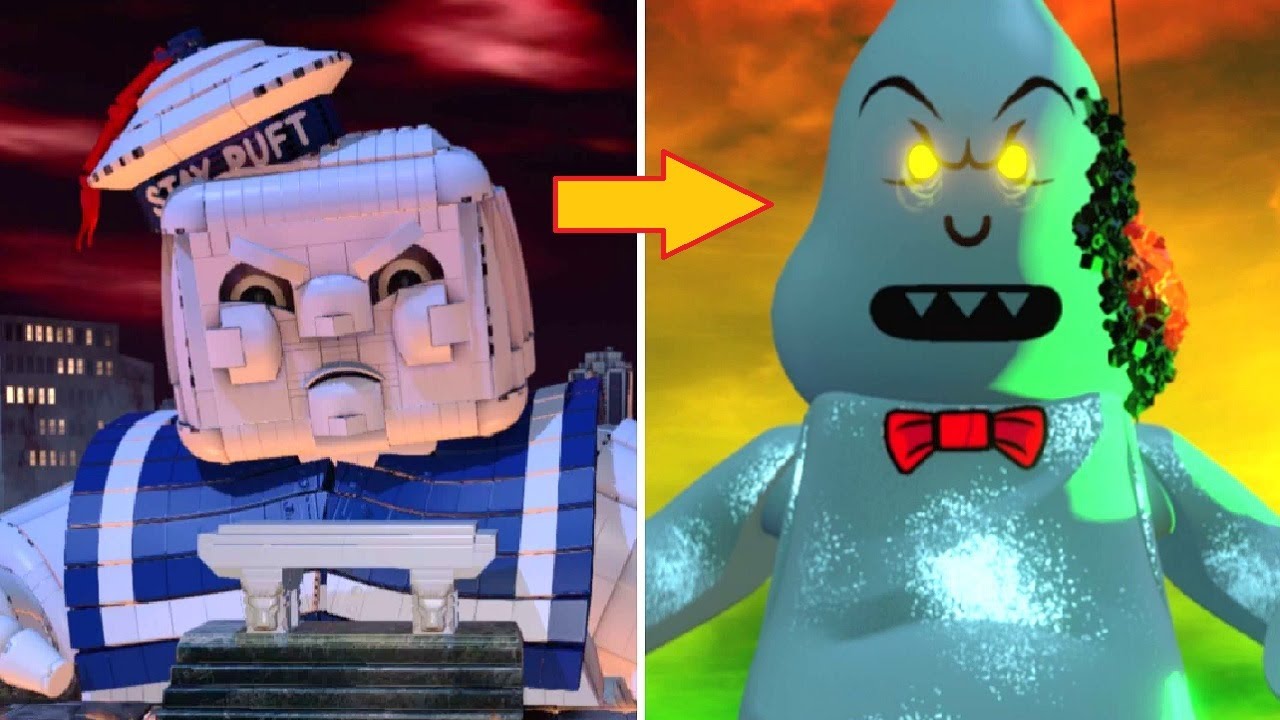The image is a composite featuring two side-by-side digital renderings of figures inspired by the Stay Puft Marshmallow Man from "Ghostbusters." On the left, there's a blockish, possibly Lego-like version of the iconic character. This figure, characterized by its white body, blue costume, and red ribbon-adorned hat, has a square, digital-rendered appearance and towers menacingly above a cityscape, reminiscent of a scene from the movie. The image on the right, connected by an arrow, presents an alternative, more grotesque interpretation of the Stay Puft character. This version is green with yellow eyes, sharp pointed teeth, and a black mouth. The body is softer, sequenced, and adorned with a red bow tie. There's some red and brown discoloration on its left side, suggesting damage or wear. The background contrasts with the yellow hues, adding to the menacing aura of the figure.